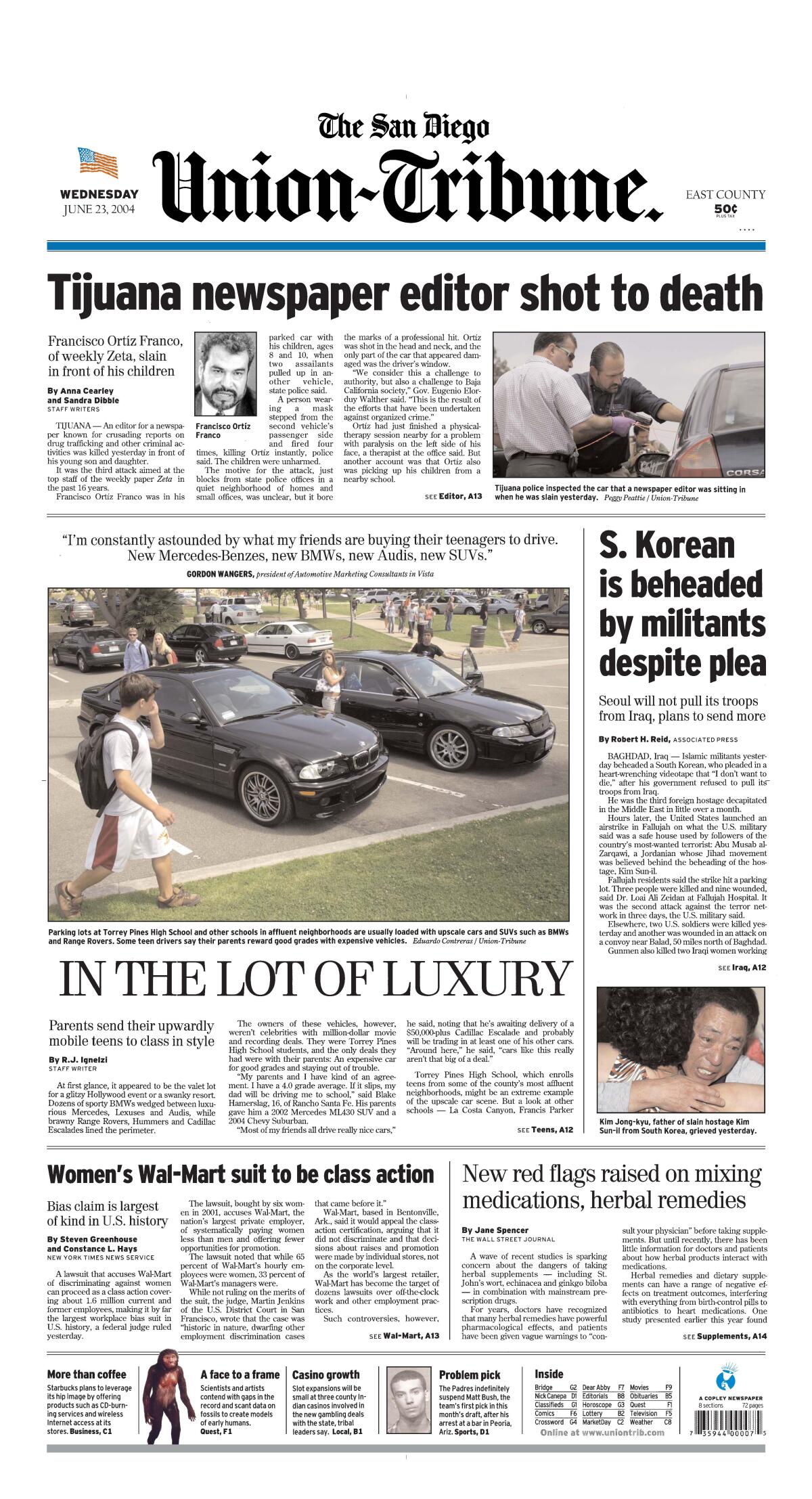The image displays the front page of the San Diego Union-Tribune dated Wednesday, June 23, 2004, with an American flag at the top left corner and a price indication of "East County, 50 cents" on the right. Dominating the page is the headline "Tijuana newspaper editor shot to death" featuring a black and white portrait of the slain editor, Francisco Ortiz Franco, and a photo of two men with guns drawn, looking into a car window. The tragic nature of the incident is highlighted by the detail that Franco was killed in front of his children. Below this, another stark headline reads "S. Korean is beheaded by militants despite plea," alongside an image of a man hugging a woman. Further down, a section titled "In the loot of luxury" discusses teenagers' purchase of Mercedes Benz cars, and there's a related image showing a man in white clothes crossing a parking lot. Additional articles at the bottom include "Woman's Walmart suit to be class action" and "New red flags raised on mixing medications, herbal remedies."